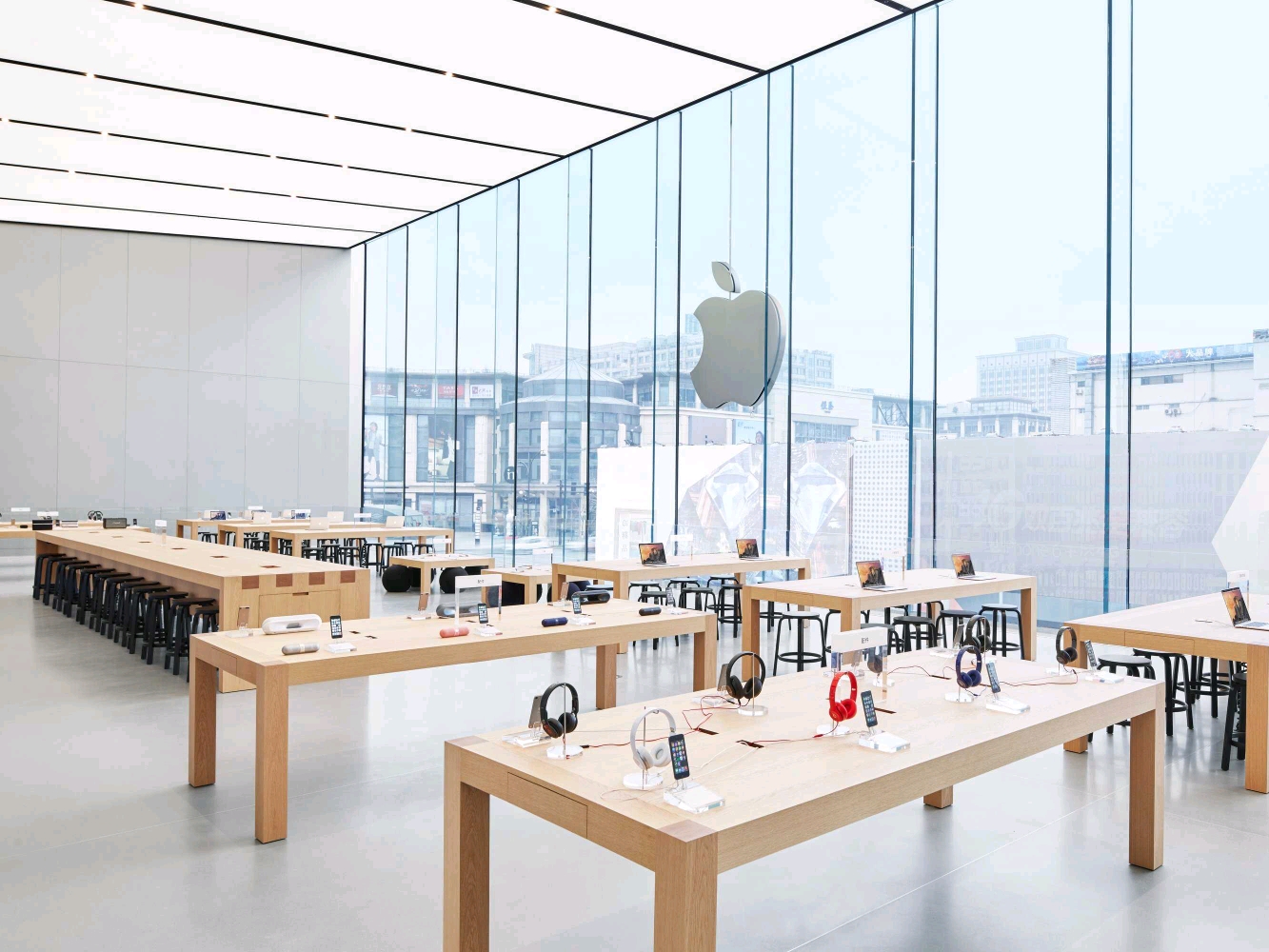The photograph captures the sleek and modern interior of an Apple Store. The ceiling features a unique design with white panels interspersed with black sections, housing embedded lights. Large glass window panes dominate the facade, offering a view of the cityscape, including what appears to be a sports stadium and various high-rise buildings. A striking gray Apple logo, illuminated brightly, is mounted on the glass.

Inside the store, the aesthetic is minimalist with white wooden tables arranged methodically. In the foreground, one table displays pairs of headphones in black, gray, blue, and red. Nearby, another table showcases a laptop. Additional tables, equipped with laptops or speakers in hues of gray, salmon, blue, and black, are spaced evenly throughout the store. Black stools accompany these tables, providing seating options for visitors. The back of the store features a few empty blonde wooden tables with more black stools.

The floor is tiled in gray and reflects the sunlight streaming through the expansive windows, adding to the bright and open atmosphere. The image quality is decent, albeit slightly pixelated toward the back of the store, ensuring most details are clearly visible.